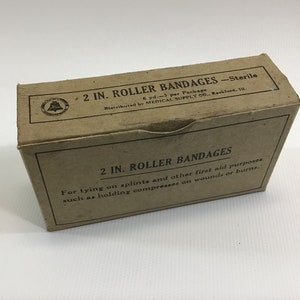The image is a small, square color photograph with a plain white background. The light source is positioned in the top right corner, casting shadows both behind and in front of the object, with the shadow predominantly visible behind it. The object in focus is a slim, light brown cardboard box typically used for containing bandages. This non-glossy, raw-textured box bears the label "Two Inch Roller Bandages, Sterile" prominently across the top.

The design includes a round seal emblem, which contains an indistinct symbol that resembles the Liberty Bell, although the details are too small to decipher clearly. The front of the box features a minimalist design with another inscription of "Two Inch Roller Bandages" and additional, smaller text that is illegible but suggests usage instructions or additional information.

A small lip or spout is present at the top of the box, presumably to facilitate easier opening by allowing a finger grip. Overall, the box exemplifies a simple and utilitarian design intended for practical use.